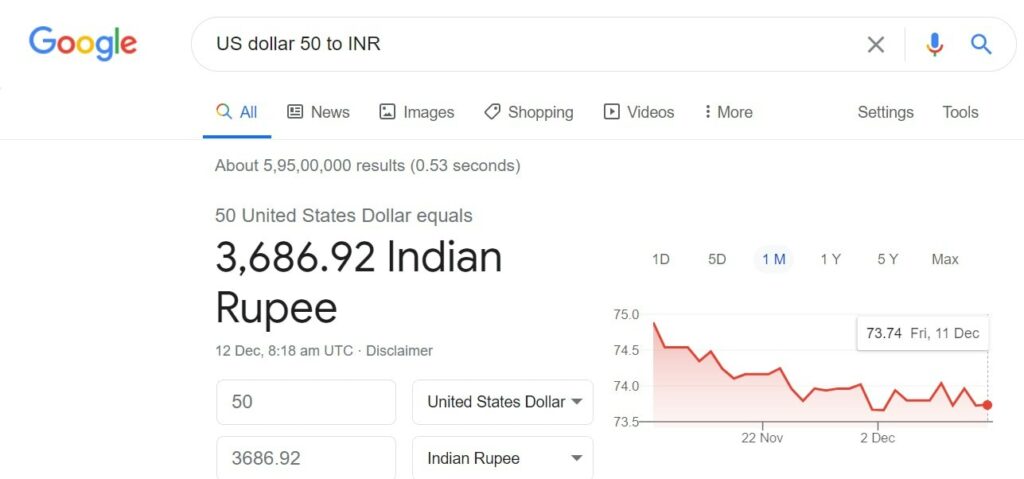A Google search result is displayed, showing the conversion rate between US dollars and Indian rupees. The search query "50 USD to INR" reveals that $50 is equivalent to 3,686.92 Indian Rupees. The image highlights an individual seeking to understand the current exchange rate between the US dollar and the Indian rupee, likely for purposes of travel, financial planning, or currency exchange.